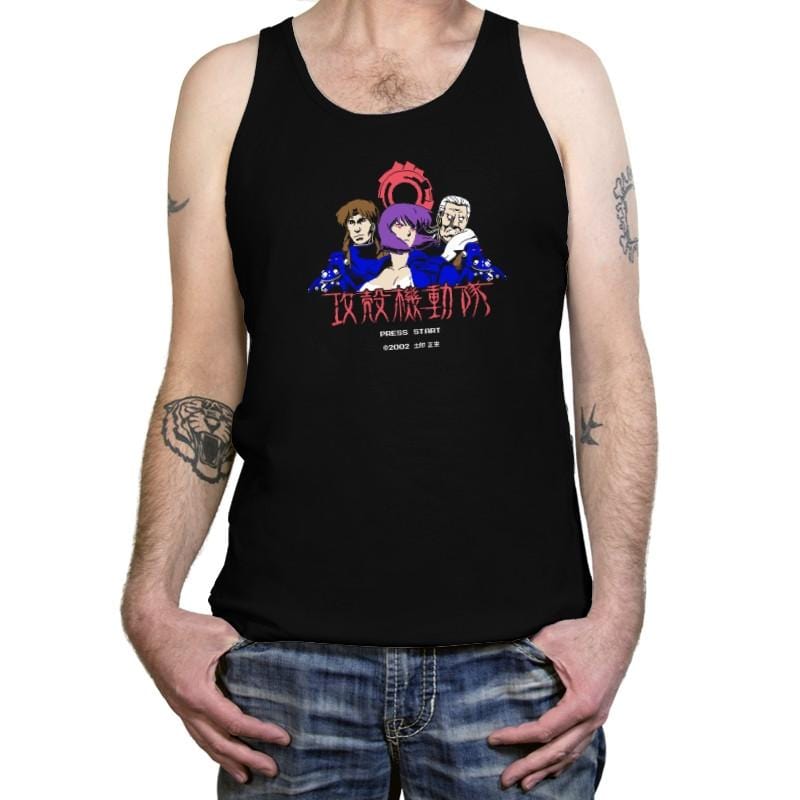The image showcases a black tank top adorned with red text, though the specific message is unreadable. Prominently displayed on the front of the tank top are two cartoon characters, both depicting Caucasian individuals with varying hair colors—one with brown hair and the other with purple. The person wearing the tank top has visibly tattooed arms, featuring intricate designs in a dark black ink. They are also wearing a pair of blue jeans, contributing to a casual and relaxed appearance. The upper part of the person is visible, though their face is not shown in the image.